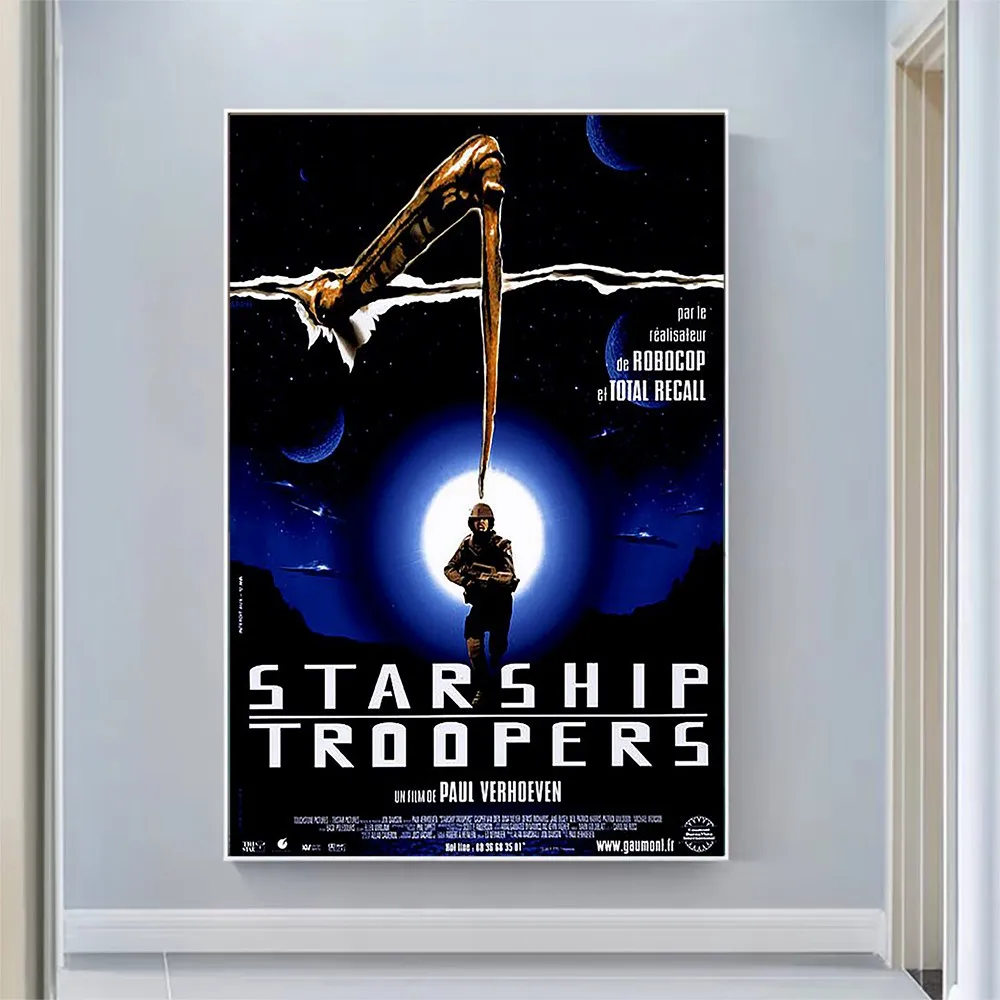This image is a color photograph capturing a very large, theater-authentic movie poster framed and mounted on a light gray wall within a home. The poster, measuring approximately 60 inches tall by 36 inches wide, is encased in a narrow silver frame, making the vibrant artwork the focal point. The poster promotes the film "Starship Troopers" and features a dark blue and black background. Central to the composition is a white, glowing moon surrounded by radiating lighter blue hues and white stars, with a metallic spaceship and a dagger-like appendage descending from its nose. Beneath this spaceship, a soldier clad in a helmet and military gear holds a rifle, which is pointed slightly to the right, with his left arm supporting the muzzle. Bold white text spans the lower third of the poster, with "Starship" and "Troopers" prominently displayed in large, all-caps font separated by a horizontal white line. The poster includes French text attributing the film to Paul Verhoeven and referencing "Robocop" and "Total Recall," along with the website "www.gaumont.fr," indicating its French origin. To the right of the poster, a white door frame leads to another room, while below the poster, a white baseboard delineates the transition from the gray wall to the gray floor.